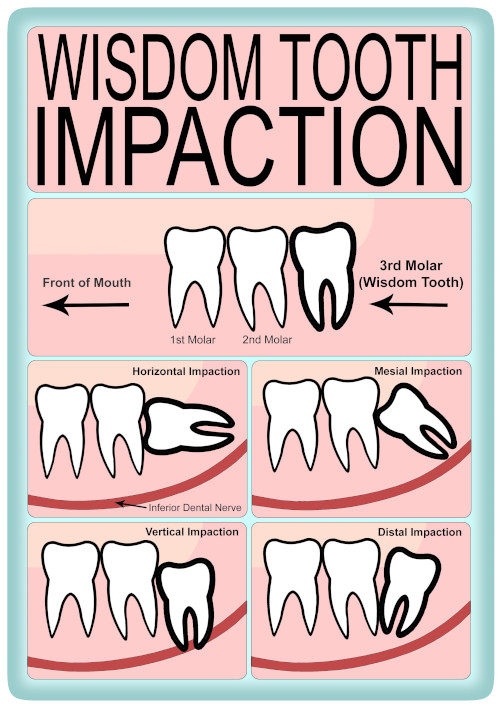The image is a detailed informational diagram likely from a dentist's office, explaining wisdom tooth impaction. It features a light blue border surrounding a pale pink background divided into several sections with thin blue lines. At the top, in large black capital letters, it reads "WISDOM TOOTH IMPACTION."

In the main section below, there’s an illustration of a mouth showing three teeth side-by-side. The leftmost tooth is labeled "First Molar," the middle tooth as "Second Molar," and the rightmost tooth, outlined in bold, is labeled "Third Molar (Wisdom Tooth)" with an arrow pointing to it. To the left of this tooth diagram, there is a label "Front of Mouth" with an arrow pointing leftwards.

Beneath this illustration, the diagram is split into four smaller sections, each depicting a different type of wisdom tooth impaction. The top left section shows a "Horizontal Impaction," where the wisdom tooth is oriented sideways against the neighboring tooth, with a red curved line labeled "Inferior Dental Nerve" beneath it. The top right section depicts a "Mesial Impaction," where the wisdom tooth is angled at about 45 degrees, pointing towards the front of the mouth with the nerve shown below. The bottom left section illustrates a "Vertical Impaction," where the wisdom tooth is pushing downward onto the nerve. Finally, the bottom right section shows a "Distal Impaction," where the wisdom tooth is angled towards the back of the mouth, with the root impacting the neighboring molar and the red nerve line beneath it.